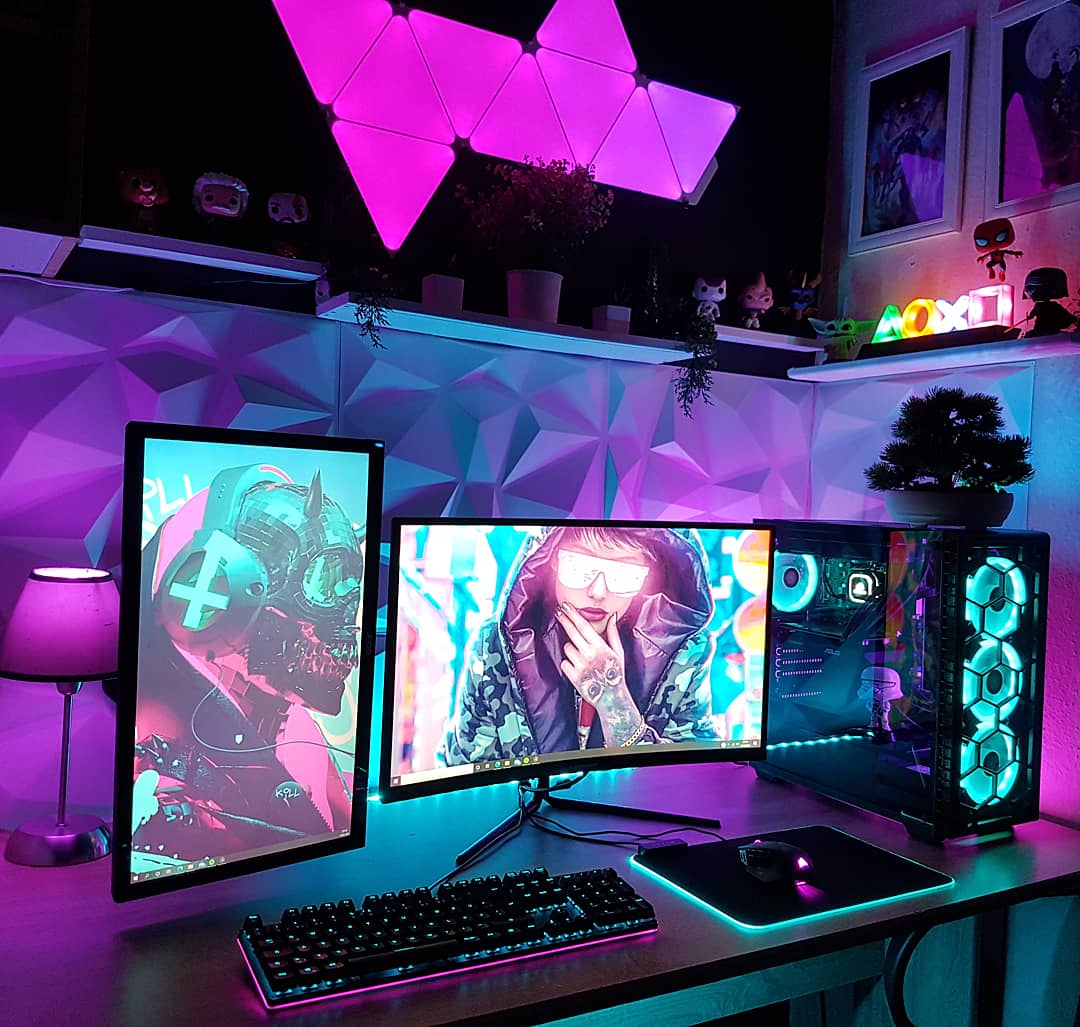The image showcases an impeccably organized gaming or streaming desk setup in what appears to be a bedroom. The desk is silver, featuring two monitors—one positioned horizontally and the other vertically. The vertical monitor is set up on the left, while both screens display vivid graphic backgrounds. A sleek black keyboard with blue LED backlighting sits in front, accompanied by a black mouse pad highlighted by outer white lights and a matching black mouse.

The right side of the desk houses a sophisticated gaming PC with a black exterior illuminated by three white lights and an overall blue glow. Purple and blue LED lighting casts a trendy ambiance across the room, enhancing the immersive atmosphere typical of a gaming or streaming environment. Above the desk, a shelf adorned with various plants, figurines, and art pieces adds personal flair to the setup. On the wall behind the monitors, framed artwork and a PlayStation logo featuring the iconic triangle, circle, X, and square symbols further emphasize the gaming theme. Additionally, a stylish desk lamp provides functional lighting against the colorful backdrop, completing the high-end, aesthetically pleasing scene. The image is of very high quality, with no people or text, ensuring the focus remains on the elaborate setup.